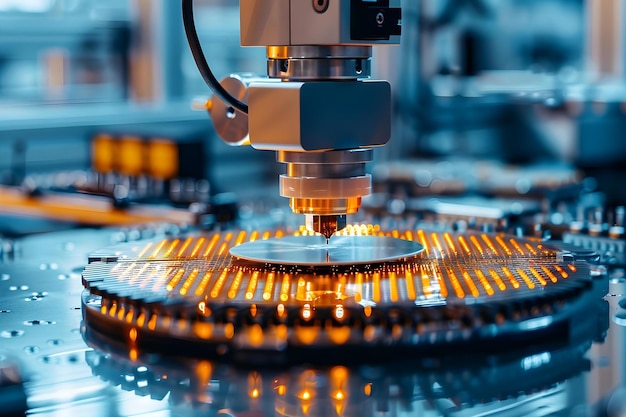The image features a highly detailed, computer-generated close-up of a rotary tool, likely part of a CNC (Computer Numeric Controlled) machine, performing a task in a machine shop. The central focus is a complex drill apparatus composed of multiple components, including a silver, finely-pointed drill tip, rectangular white shapes, and silver discs. Surrounding the drill are thin flat silver discs and a larger circular black structure illuminated by orange lights on both sides. Below this assembly is a reflective, glass-like surface with bluish hues to the left. The machine shop background is blurred, scattered with additional machinery and orange and light blue tones, adding to the industrial ambiance. The image appears slightly surreal, with some elements like water droplets or blurriness suggesting it's a computer-generated depiction rather than a real photo.